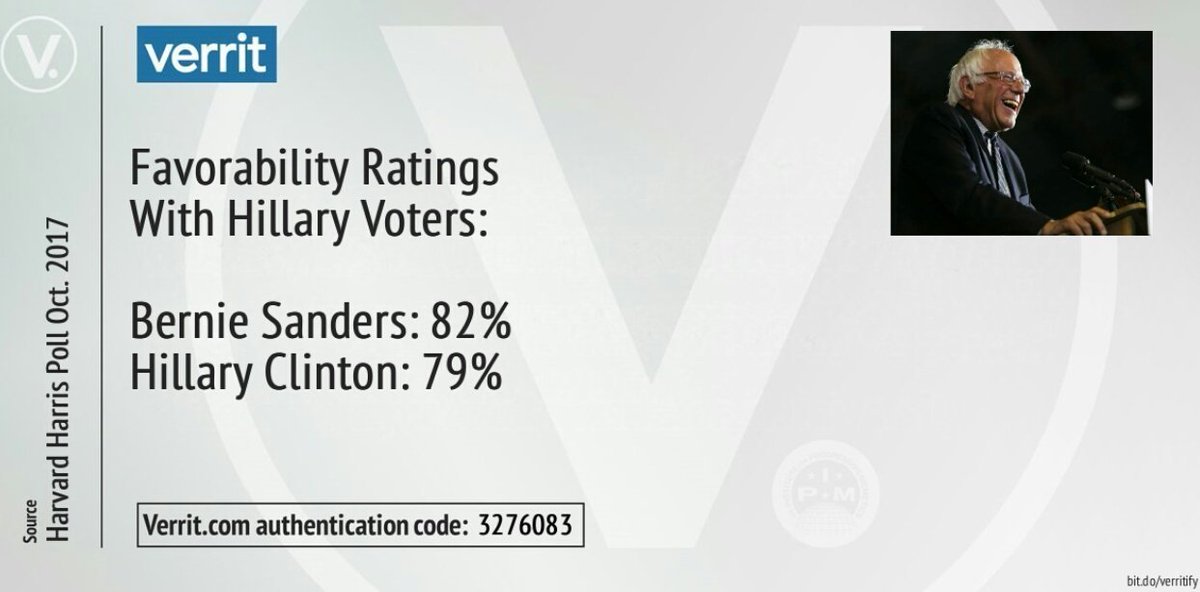A Verit.com authentication code slip, based on a Harvard-Harris poll from October 2017, details favorability ratings among Hillary Clinton voters. The card prominently features two Verit logos: one with a "V." encircled and reversed out of a gray background to white, and a blue band displaying "verit" in lowercase with the text reversed out to white. The slip reveals that Bernie Sanders holds an 82% favorability rating, compared to Hillary Clinton's 79%, among these voters. On the right side of the slip, there is a photograph of Bernie Sanders. The bottom of the card includes the Verit.com authentication code: 327-6083. This slip appears to be a product from Verit, an organization that might be involved in polling.